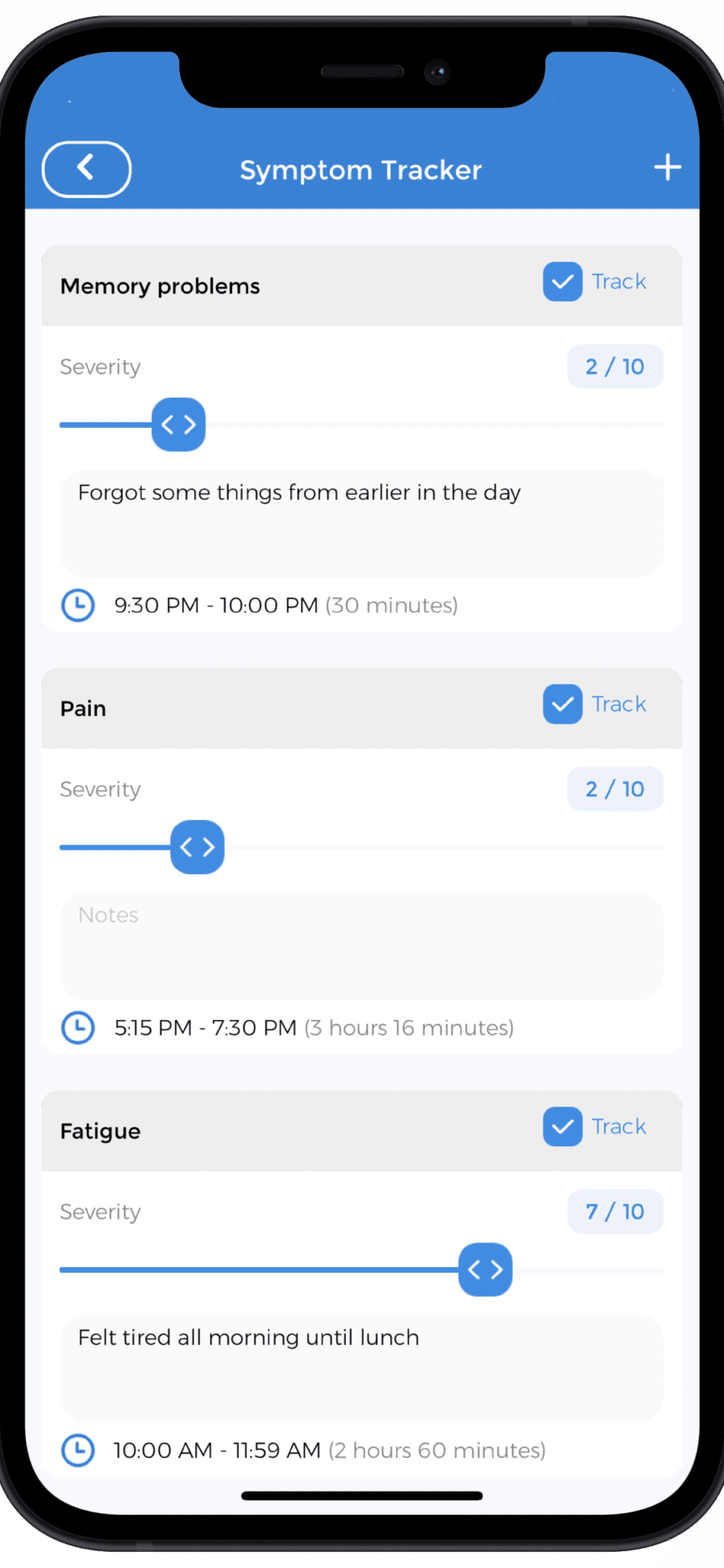This image is a screenshot of a cell phone displaying a health tracking app. The cell phone has a black border and a white screen. At the top of the screen, a blue banner is visible, displaying the title "Symptom Tracker" in white text, flanked by a back arrow on the left and a plus sign on the right.

Below the blue banner, there are three light gray banners with black text, each representing a different symptom category: memory problems, pain, and fatigue. Each banner features a checkbox on the left and the word "Track" on the right.

Under the "Memory Problems" category, there is a sliding scale for severity, adjustable using two arrows. The severity for memory problems is set to 2 out of 10. Beneath this scale, there is a text box where the user has entered, "Forgot some things from earlier in the day." The time period for this entry is stated as 9:30 PM to 10:00 PM.

The "Pain" category follows the same format, with the severity also rated at 2 out of 10 on the sliding scale.

Under the "Fatigue" category, there is another sliding scale where the severity is rated much higher, at 7 out of 10. In the associated text box, the user has written, "Felt tired all morning until lunch."

Overall, the screenshot provides a detailed view of the user’s entries for tracking their symptoms of memory problems, pain, and fatigue using the app's interface.